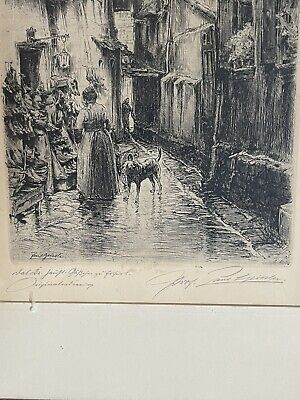This image features a meticulously detailed, black ink drawing on a now slightly brownish, aged white cardstock, resembling an old ink drawing or a vintage postcard. The scene captures a narrow cobblestone street, evoking a nostalgic ambiance of old Ireland or Europe, with a woman in a long, late 1800s to early 1900s style dress. Her hair, pinned up, accentuates her timeless elegance as she stands with her faithful dog by her side. She appears to be looking away towards a produce stand, perhaps part of a bustling farmer's market located to the left in this quaint alleyway. The intricate details include a narrow alley with the shadow of another person, and a window adorned with flowers on the right side, lending charm to the surroundings. The dog, standing by her right leg with its tail held high, suggests a moment of contentment. The image is signed at the bottom in an ornate script, though it is faint and difficult to read. The entire scene exudes a sense of serenity and historical charm, encapsulating a moment in time through the delicate artistry of the period.